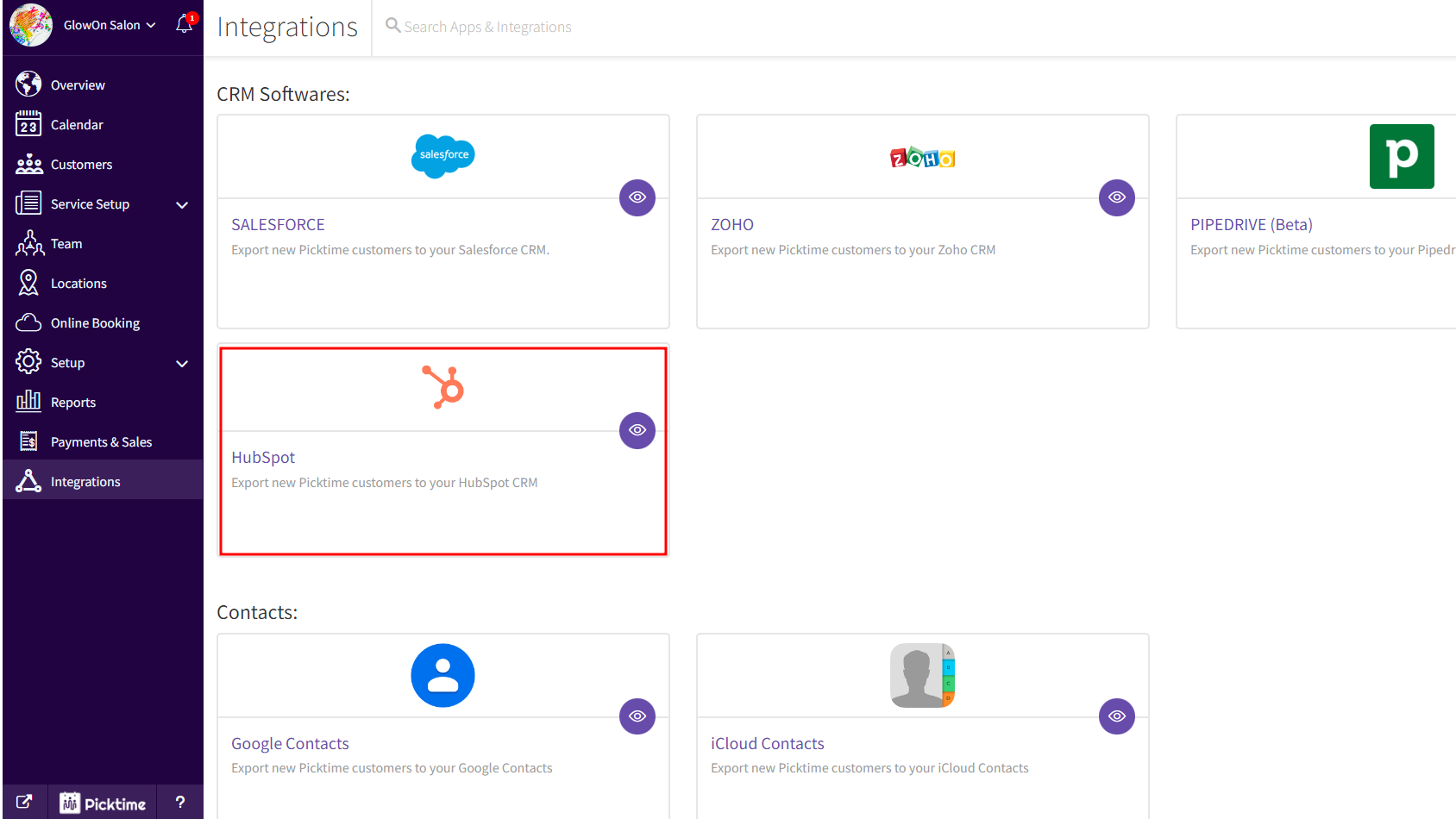This image is a cropped screenshot of the PicTime application interface, showcasing its Integrations panel. The left panel, which is notably narrow and dark blue, features the PicTime logo prominently in the bottom left corner. At the top of this panel, the user's profile picture and name are displayed, accompanied by a drop-down menu for switching users. An alert icon with a red notification dot is visible in the far right at the top, indicating that there are pending alerts. 

The left panel also contains a vertical list of options, with 'Integrations' highlighted at the bottom. The main section of the page, which has a white background, focuses on integrations and is titled "Integrations" in large gray letters at the top left. Adjacent to this title is a search bar for easy navigation. Below the search bar, another heading, "CRM Softwares," is displayed in large gray letters. The section features four boxes representing different CRM software applications, with HubSpot selected and highlighted by a red border.